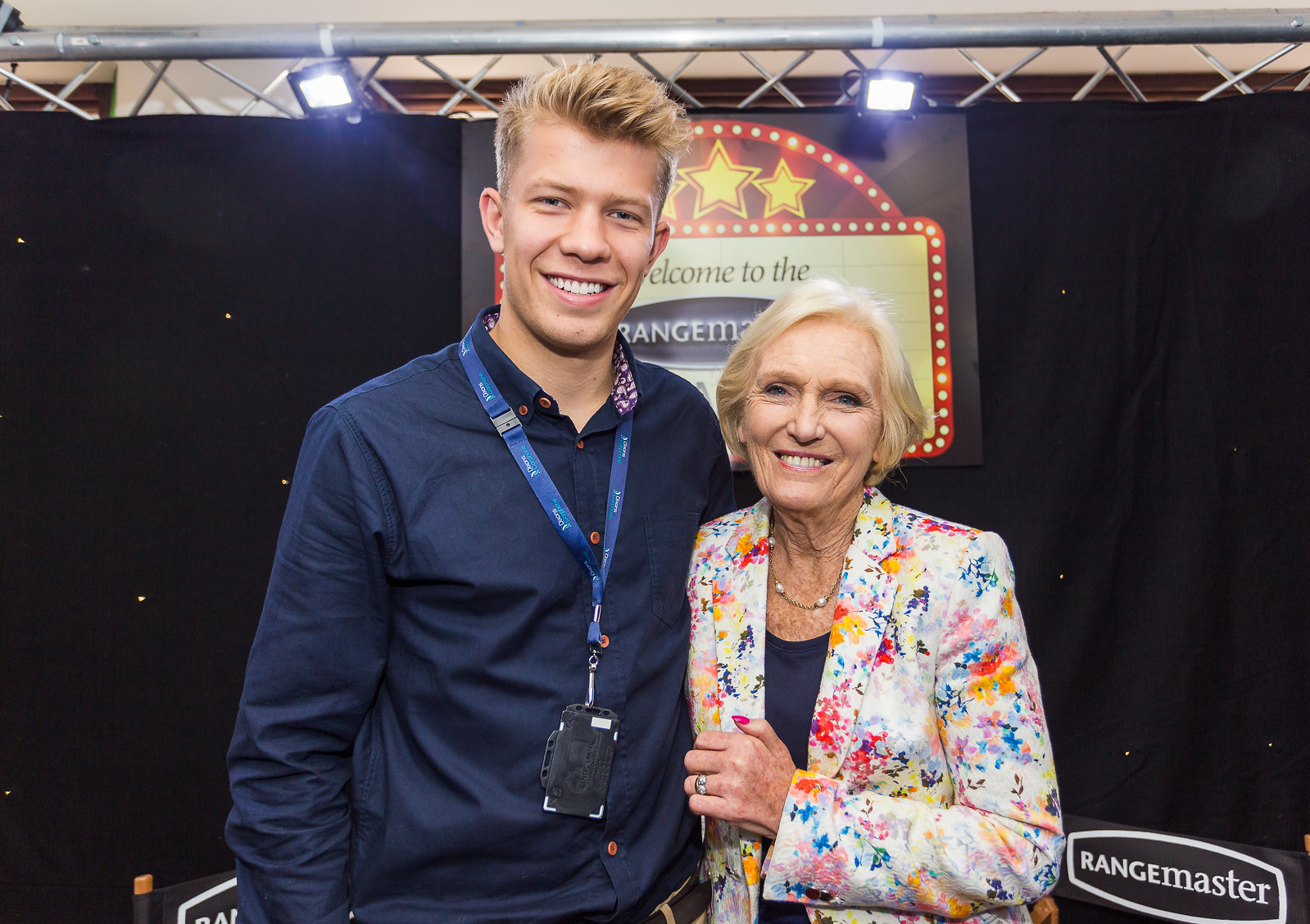The horizontal rectangular photograph captures a young man and an older woman standing closely together, posing and smiling for the camera, likely at a booth in a trade show or fair. Both are white, with the man on the left wearing a dark blue button-down shirt and a lanyard around his neck, though his ID badge is obscured. He has short blonde hair and is smiling directly at the camera. The woman stands to his right and is notably shorter; she appears to be in her 50s or 60s. She is dressed in a striking floral or multicolored blazer over a blue top, accessorized with a small pearl and gold necklace. Behind them, a black curtain serves as a backdrop with a sign in the middle that reads "Welcome to the Rangemaster," accompanied by red lights and three stars at the top. In the lower right corner of the image, the brand name "Rangemaster" is also visible. Both subjects exude a sense of accomplishment and camaraderie, hinting at a recent achievement or successful event.